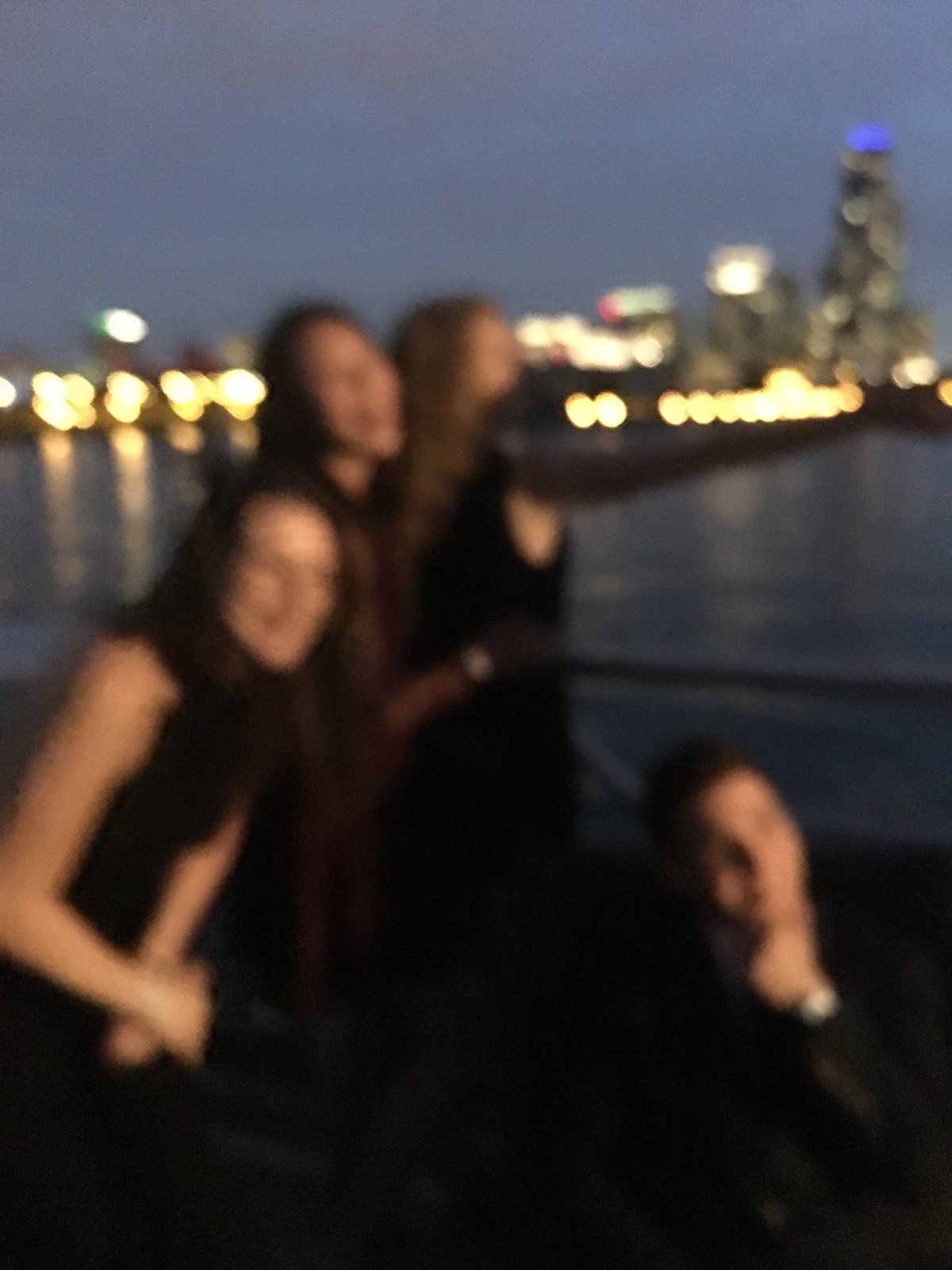In this extremely blurry nighttime photo, four individuals, all Caucasians with brunette hair, are posing by what appears to be a waterfront. The group consists of three women standing side by side to the left and a man crouched down to the right, his fist under his chin, facing forward but looking off to his right. All four are dressed in dark black clothing, with the man notably wearing a black suit and a blue button-up shirt. The women have shoulder-length hair and seem to be smiling despite the blur. Behind them is a dimly lit harbor with a blue body of water and an array of distant lights, suggesting a cityscape with a few skyscrapers. The sky above is a dark grayish-blue, adding to the nighttime setting. The ground they are standing on appears to be black.